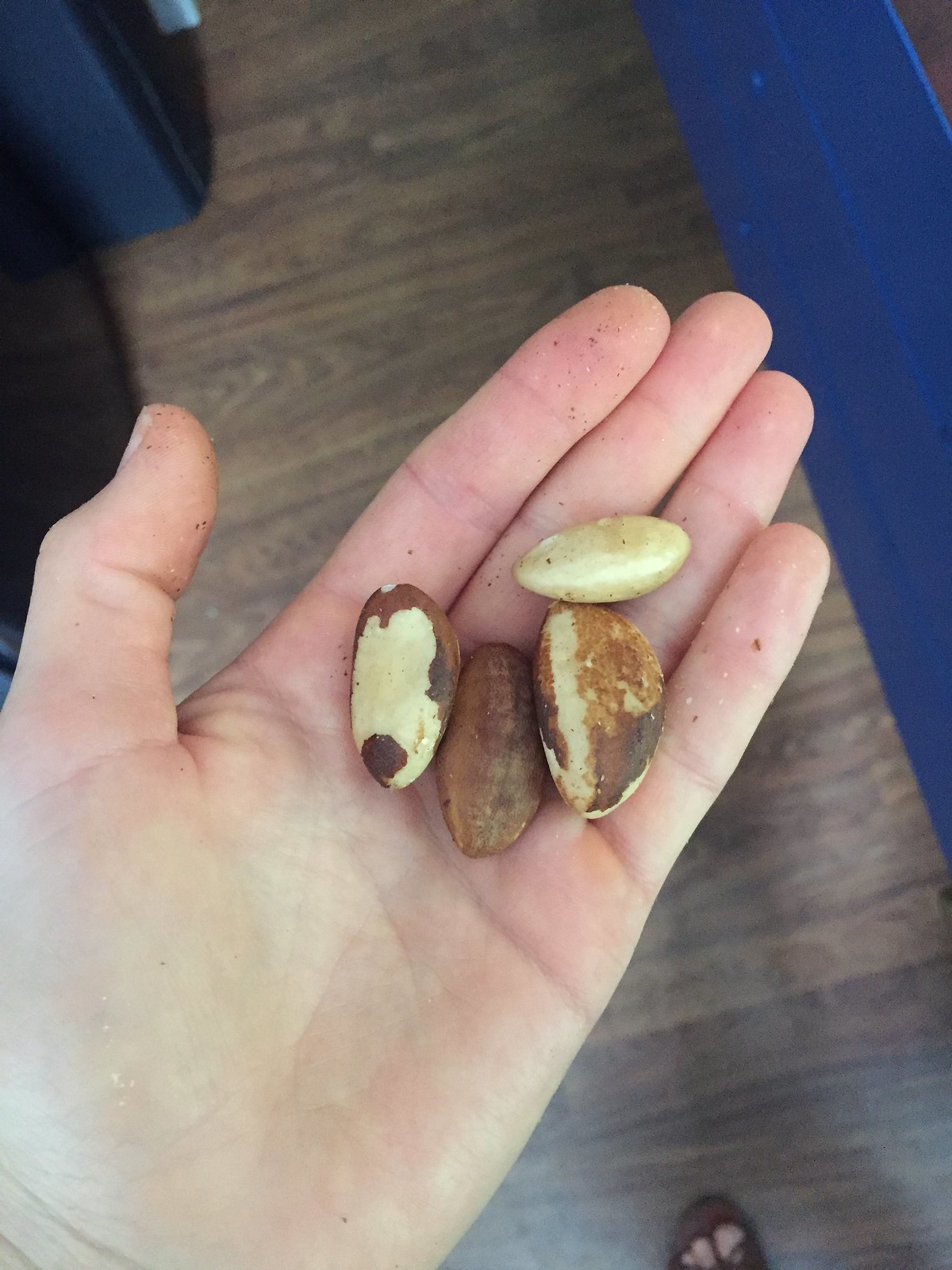The photograph captures a detailed, close-up view of a left hand, palm up, holding four distinct nuts of varying sizes and colors. These nuts are most likely walnuts, though there's some speculation they could be Brazil nuts or almonds based on their textures and appearances. Three of the nuts have a rough, dark brown exterior typical of walnuts, while the fourth, located at the top right of the hand, features a lighter and smoother surface, potentially indicating a different type of nut. The person holding the nuts has fair, pale skin. Just below the hand, in the bottom right corner, a foot clad in a sandal is visible, with its toes peeking out. The backdrop includes a synthetic wood floor, often found in boats or confined spaces, and a blue baseboard on the right side of the image. Overall, the photo's main focus is the hand presenting the four diverse nuts.